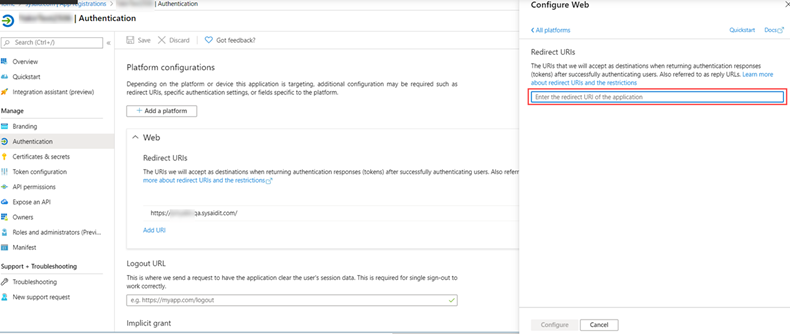The image captures an application's settings screen, characterized by a detailed layout. On the left side, the vertical menu displays various sections starting with "Overview," "Quick start," and "Integration assistant," under a primary category labeled "Manage." Directly below this category are additional options: "Branding," "Authentication," "Certificates and secrets," "Token configuration," "API permissions," "Expose an API," "Owners," and "Roles and administrators." The bottom section lists "Support and troubleshooting." Notably, beneath the "Authentication" label is a blurred-out image. 

To the right, in the main content area of the screen, the focus is on the "Platform configurations" section. Prominently featured is an "Add platform" button. Below this, a "Web" category is displayed, which includes options for "Redirect URLs." Further to the right within this menu window is a detailed "Configure web" pane, presumably offering specific settings for web platform configurations. The overall layout is designed to provide a comprehensive array of configuration options for the application.